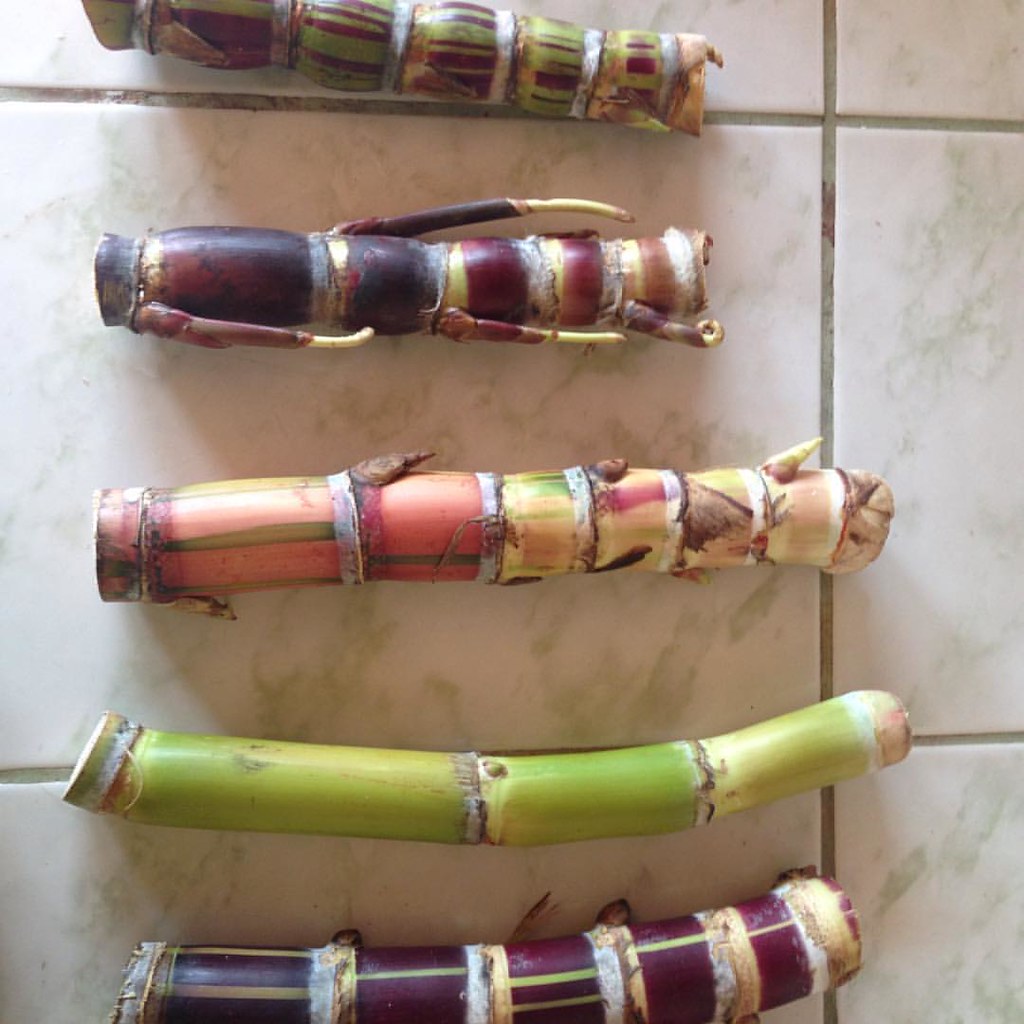The photograph showcases a series of five vividly colored stalks that resemble bamboo, arranged on a white tile surface adorned with gray marbling and visible grout lines. Each stalk varies in hue and pattern, contributing to a striking visual display. The bottom stalk is predominantly purple, followed by a green stalk. The third one features a mix of pink and green, while the fourth is another shade of purple combined with green. The topmost stalk, primarily deep red with hints of green, appears slightly curved. All the stalks are segmented with distinct rings around their circumference and have a hard appearance. Despite their artistic and vibrant presentation, their exact nature remains uncertain. Additionally, the tile surface features a noticeable burgundy stain, adding to the photograph’s intricate details.